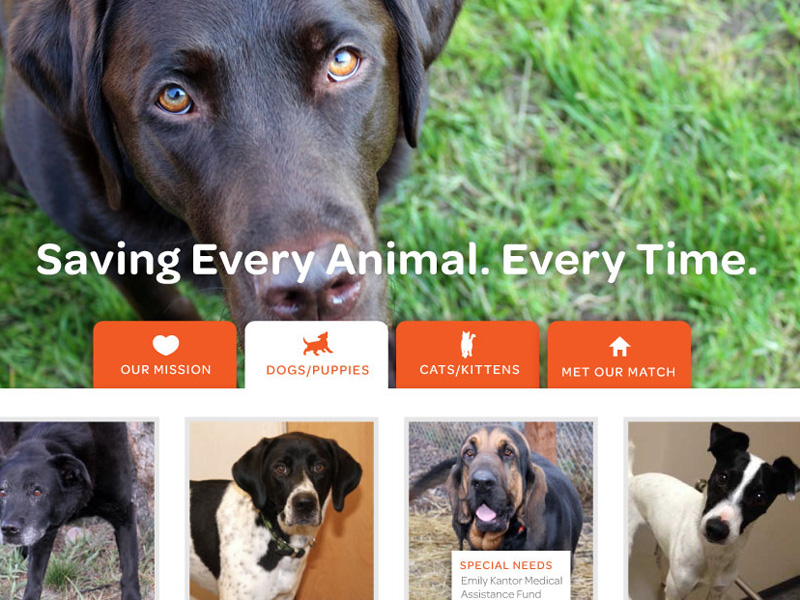Screenshot of ASPCA Website: A poignant close-up of a black dog with soulful brown eyes dominates the top of the page, reflecting a somber expression as it gazes directly into the camera. The blurred background of green grass contrasts the sharp focus on the dog, underlining its prominence and evoking a sense of urgent compassion. Above the image, in a bold white font, is the phrase "Saving Every Animal Every Time," encapsulating the organization's mission.

Below this powerful image are four navigational tabs. The first one, with an orange background and a white heart, reads "Our Mission" in white text. The second tab, selected with a white background, is labeled "Dogs and Puppies," indicating the section currently viewed. The third tab, also orange, is labeled "Cats and Kittens." The fourth and final tab, similarly orange, states "Meet Our Match."

At the bottom of the screenshot are four additional close-up photos of dogs: 

1. A black dog on the far left.
2. A black-and-white dog next to it, characterized by black ears and head with a predominantly white or light gray body.
3. A dog with a mix of brown and black fur on its face, accompanied by a caption that reads "Special Needs: Emily Cantor Medical Assistance Fund."
4. The dog on the far right has a white body with a unique fur pattern—white down the center of its face, with black fur covering the ears and sides.

This screenshot captures the essence of ASPCA's commitment to rescuing and caring for animals, subtly reflecting their recognizable branding and empathetic outreach.